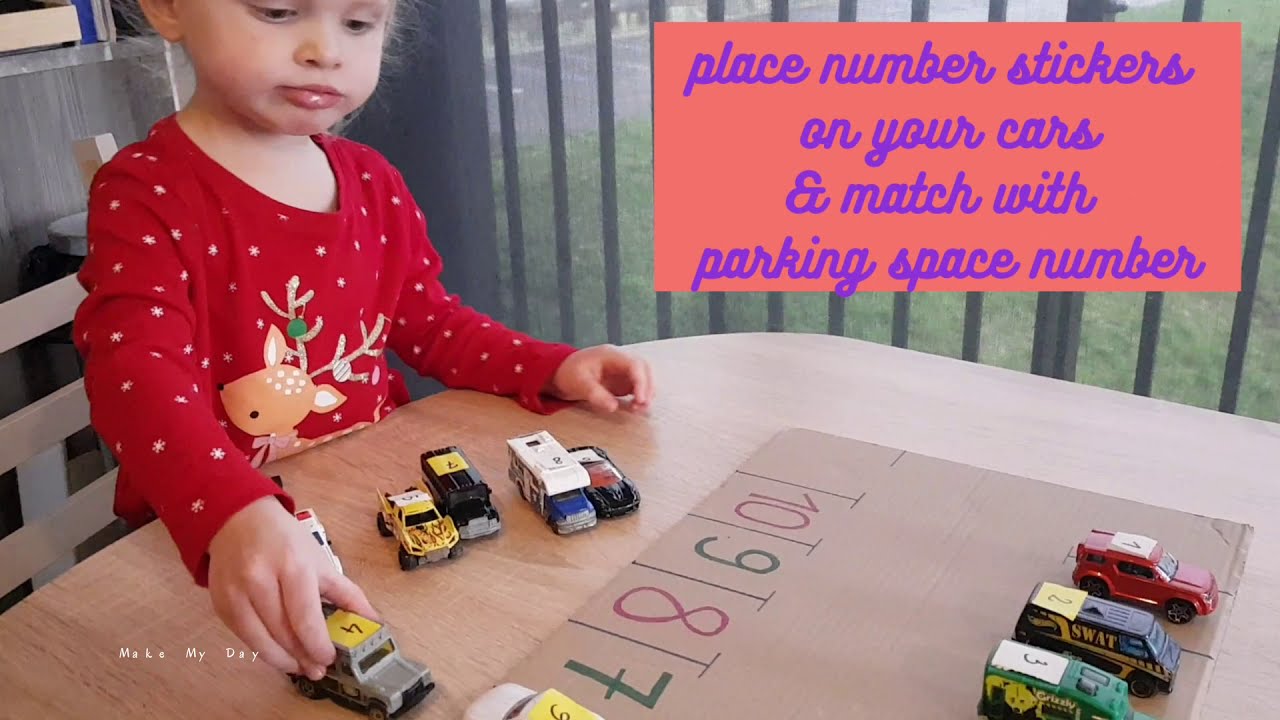In an indoor setting flooded with natural light, a young blonde-haired girl sits at a wooden table engrossed in playing with her collection of multicolored toy cars. Dressed in a festive red long-sleeve shirt adorned with a reindeer, she arranges the cars—vans, trucks, a bus, and a sleek black Ferrari—on a cardboard layout that mimics a parking lot. This cardboard is meticulously numbered 10-9-8-7, guiding the placement of each vehicle. A pink and purple box in the upper right corner bears the text, "Place number stickers on your cars that match with parking space number," offering playful instructions for her activity. Behind her, the room features a white chair and a gray railing visible through the window, revealing a green-streaked outdoor view of a street and parking lot. The ambiance suggests a living room or kitchen setting, perhaps even a streaming scene where she demonstrates her imaginative play.